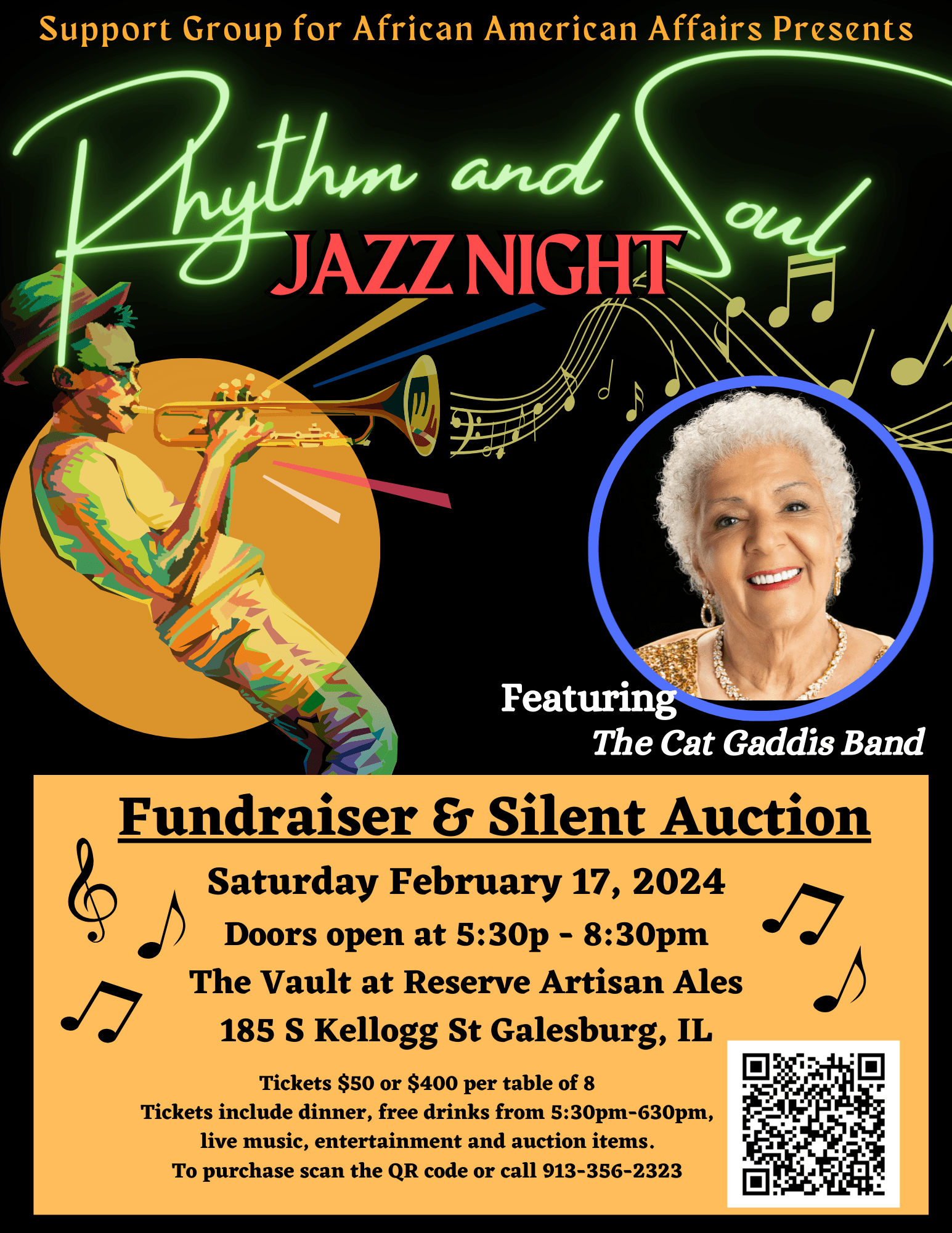The poster for the Rhythm and Soul Jazz Night, a fundraiser and silent auction, features a predominantly black background with distinct sections of vibrant text and visuals. At the top, in yellow text, it reads "Support Group for African American Affairs Presents." Below, "Rhythm and Soul" is boldly displayed in green and red fonts, followed by "Jazz Night" in fluorescent blue and pink letters. Central to the poster is a blue-circled photograph of an elderly African American woman with short, curly, gray hair, smiling and wearing earrings along with a gold diamond necklace—presumably Cat Gatis. To the left of her image is a colorful cartoon of a man playing a trumpet or trombone with musical notes emanating from the instrument, set within a green circle. Detailed at the bottom, inside a gold rectangle, are the event specifics: "Fundraiser and Silent Auction, February 17, 2024, Doors open at 5:30 PM at Kellogg, Galesburg, Illinois." The ticket prices are listed as $50 per person or $400 for a table of eight. The poster also highlights that the event features live music by the Cat Gatis Band.